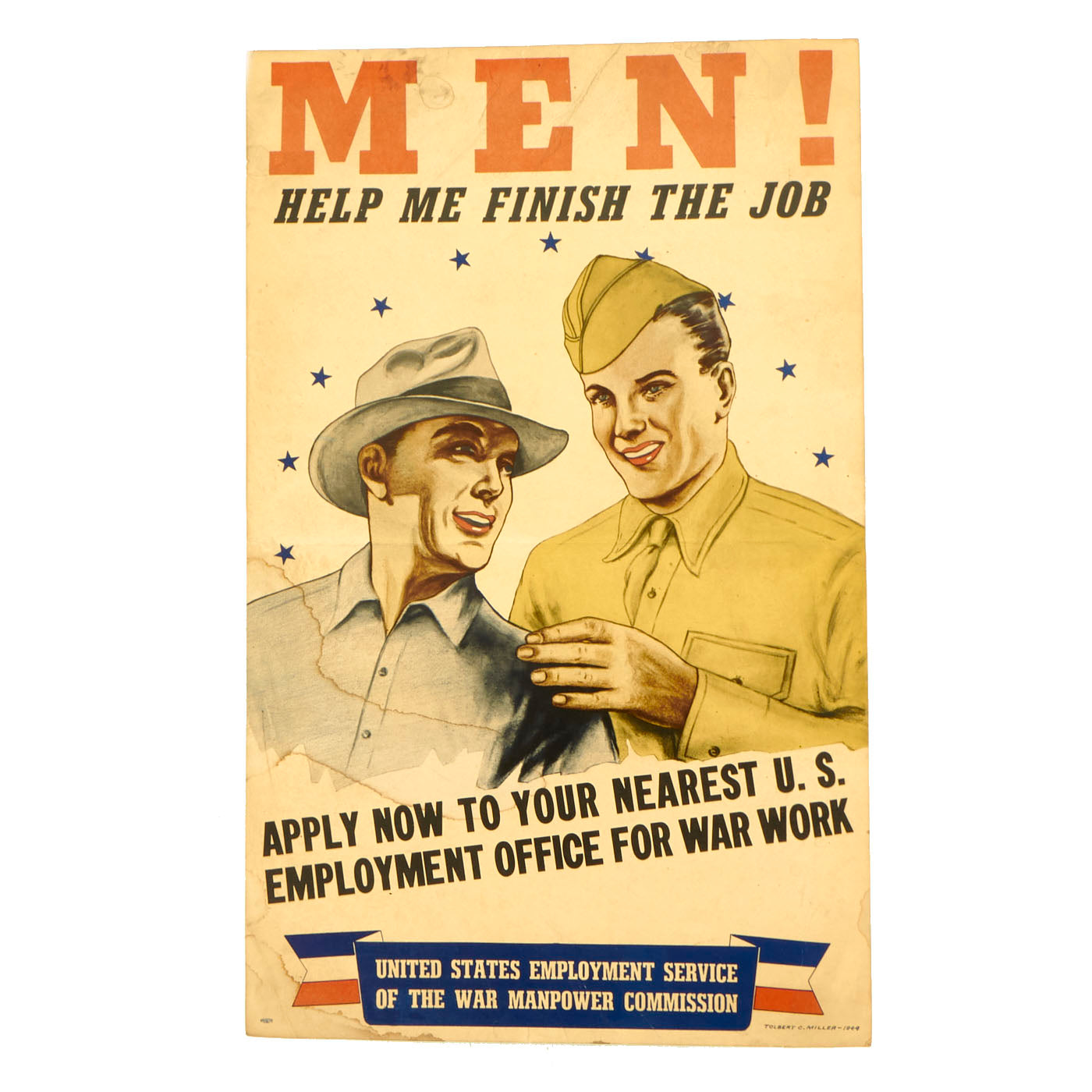This vintage World War II recruitment poster features a beige background with large, spaced-apart, dull orange-red letters at the top spelling "MEN!" Below, in smaller black capital letters, it reads, "HELP ME FINISH THIS JOB." The central image depicts two smiling Caucasian men. The man on the right, dressed in a light green military uniform with a hat, places his left hand on the shoulder of the man beside him. The other man wears a blue button-down shirt and a white hat with a black band. Blue stars form an arc above the men's heads, adding a patriotic touch. Diagonally across the bottom, in black capital letters, it says "APPLY NOW TO YOUR NEAREST U.S. EMPLOYMENT OFFICE FOR WAR WORK." Beneath this text, within a blue rectangle flanked by red, white, and blue banner-like ribbons, it reads "UNITED STATES EMPLOYMENT SERVICE OF THE WAR MANPOWER COMMISSION." The poster radiates a sense of camaraderie and patriotic duty, urging viewers to join the war effort.